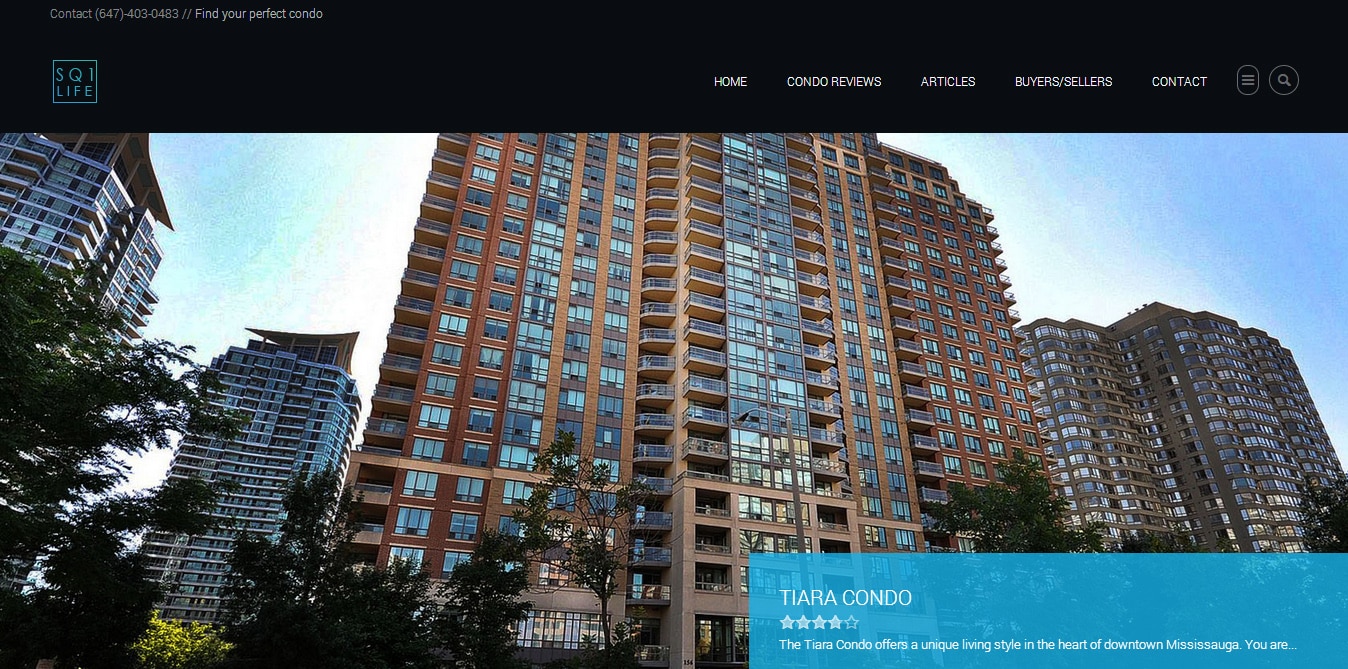The image is a horizontal rectangle with the top quarter filled with a solid black color, which stretches from left to right and contains some difficult-to-read text. This text appears to be in a turquoise square, displaying "SQ1" followed by "LIFE" in smaller letters beneath it. Scanning from the midpoint to the right edge of the black section, we see several white, all-capitalized words: "HOME," an unreadable word, "ARTICLES," another unclear word, and "CONTACT."

The main visual content features a view of several apartment buildings, captured from a slightly low angle, making the buildings appear tall, with some cut off by the black top edge. The backdrop includes a vibrant blue sky adorned with scattered white clouds. Trees are visible in the upper left, lower left, and lower right corners of the image.

In the bottom right corner, a turquoise horizontal rectangle overlay contains white text that reads "Tiara Condo." Four out of five stars are filled in white next to the name. The description below states, "The Tiara Condo offers a unique living style in the heart of downtown," trailing off with "You are..." indicating there's more text not fully visible.